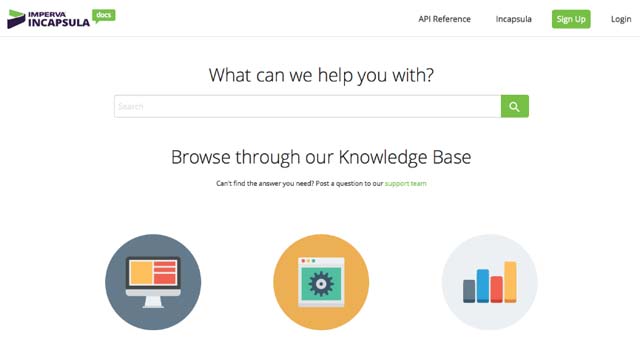The image features a clean, white background. In the top-left corner, the text "Impeva Encapsula, DOCS" is displayed, with "DOCS" in white against a green backdrop. "Impeva Encapsula" is written in purple, accompanied by a logo to its left. The logo is shaped like a "V" facing left, colored green on the top half and purple on the bottom half. 

In the upper-right corner are navigation tabs labeled "API Reference" and "Encapsula," followed by a green "Sign Up" button and a "Log In" button.

At the bottom of the image, in black text, it asks, "What can we help you with?" Below this question is a search box featuring a green search icon. Under the search box, additional text encourages users to "Browse through our knowledge base," and suggests that if the answer isn't found, they can "post a question to our support team," with "support team" highlighted in green.

At the very bottom, there are three distinctive circles. Starting from the right, the first circle is grey with a background featuring four colored bars—grey, blue, red, and orange. The icon in its center is an orange circle. The second icon shows a gear lever with a green background; the gear lever itself is grey. On the far left, the background is a slightly dark blue, containing an image of an Apple Mac computer with an orange and red screen.